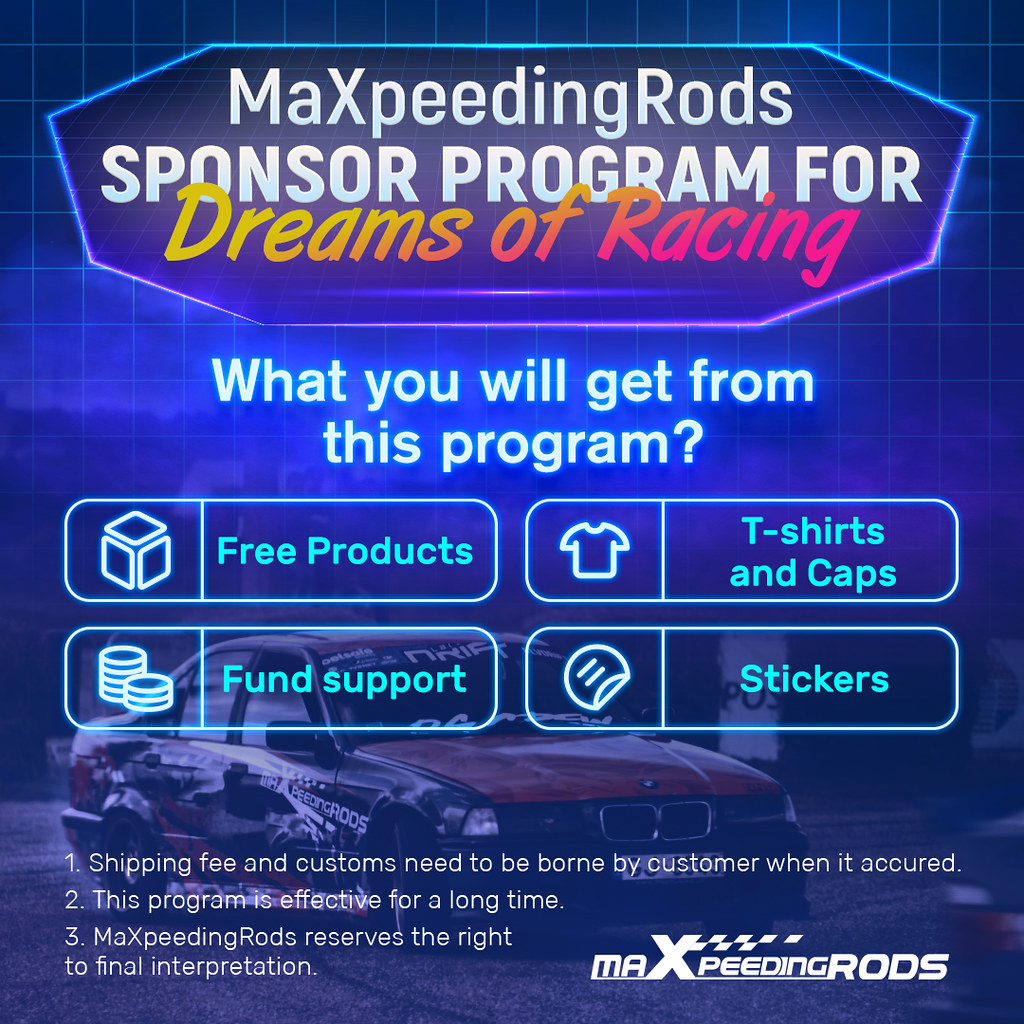This detailed square image features a digital advertisement with a dark blue, neon-like grid background, complementing a white squarish outline. At the top, a hexagonal-shaped banner with a light blue grid contains the text "Max Speeding Rods Sponsor Program for Dreams of Racing." The words "Max Speeding Rods" are styled in plain white with a silver sheen, while "Dreams of Racing" is highlighted in shades of yellow, orange, pink, and red. Below this header, the tagline "What You Will Get From This Program" is displayed in neon white font with a blue glow.

Central to the image is a purple-tinted photograph of a luxurious red race car, angled diagonally towards the bottom right of the frame. Beneath the tagline, four tabs list out the program's offerings: the top left tab features a cube icon with the label "Free Products" in blue font; the bottom left tab, displaying a coin icon, reads "Fund Support"; the top right tab shows a t-shirt icon with "T-Shirts and Caps"; and the bottom right tab, with a sticker icon, is labeled "Stickers."

Additional program details are noted at the bottom of the image: "Shipping fee and customs need to be borne by the customer when it occurs," "This program is effective for a long time," and "Max Speeding Rods reserves the right to final intervention." The Max Speeding Rods logo is also present in the bottom right corner.